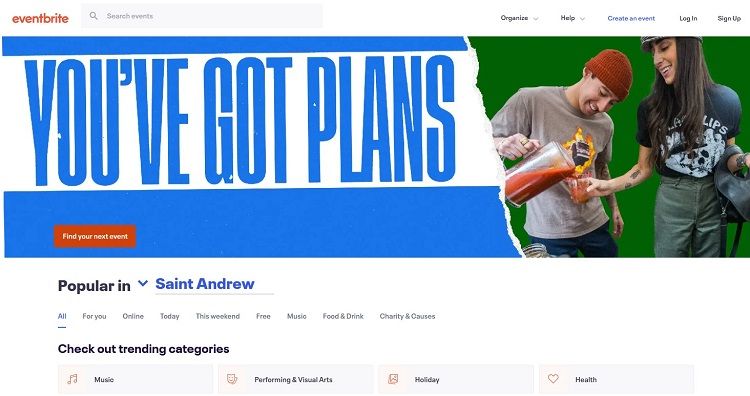This image showcases a screenshot of the Eventbrite website. The layout features a top section with a white background. Below that is a blue strip running two-thirds across the page. Following the blue strip is a segment of white, then another two-inch wide blue strip, and a final white section extending downwards. The rightmost third of the page is bordered in green.

In the top left corner, the "Eventbrite" logo is prominently displayed. Adjacent to it is a search bar. On the top right, navigation options include "Sign Out," "Log In," "Create an Event," and "Help Organize," positioned directly above the green border.

In the central section of the page, a photograph features two people. On the left is a man wearing a dark red beanie, smiling as he pours a red liquid from a pitcher into a glass positioned at his waist level. He is dressed in a gray shirt. Next to him, on the right, is a woman with long, dark hair that reaches almost to her waist. She is smiling broadly and is dressed in a black shirt and gray pants. Her right arm is bent at the elbow, assisting the man by holding the glass in front of him. She also carries a black purse over her other arm.

To the left of the image, within the white section, bold capital letters declare, "YOU'VE GOT PLANS." Below this phrase, within the blue border, is an orange tab marked "Find Your Next Event" in white text. Underneath the tab, in black text, it reads "Popular," followed by "St. Andrew" in blue. There are 10 icons representing various categories such as food, drink, music, free events, weekend happenings, and more.

Additionally, there is a section titled "Check Out Trends" listing categories including "Music," "Performing & Visual Arts," "Holiday," and "Health."